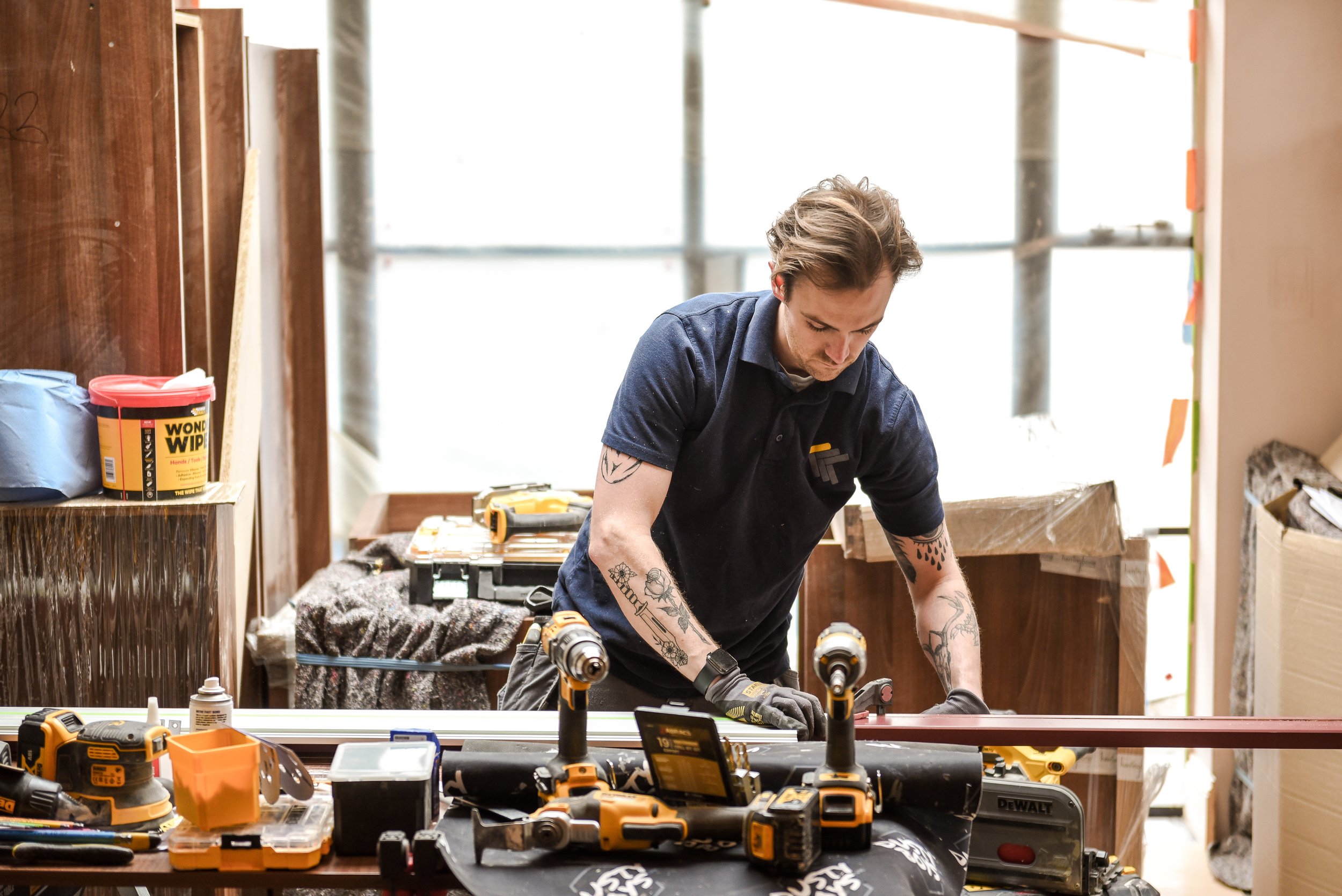The photograph captures a realistic scene of a workshop, likely a carpentry or woodshop. Horizontally oriented, the image centers on a white male in his 20s or 30s, with blondish-brown hair swept back and black stubble on his face. He stands at a work table covered in various tools, including orange and black drills, sanders, and a yellow and red bucket. The man is wearing a dark blue short-sleeved collared shirt with an orange spot near the pocket area, and black gloves. His forearms and upper arms are adorned with black ink tattoos, including images of a knife, a rose, and raindrops. 

In the background, a large white window with black frames segmented into nine sections allows light to flood the room. To the left of the frame, a radiator with labeling or a sticker can be seen, and a wooden wall contrasts with the beige drywall on the right. The table in front of him holds a long piece of wood with parts stained brown and others left in their natural light tan state. The man appears to be deeply focused on his task, looking down as he works with a tool, likely a saw, on the piece of wood. Additional materials such as containers of implements, a bucket, and tape can be seen scattered around the workspace, completing the busy and industrious atmosphere of the carpentry shop.